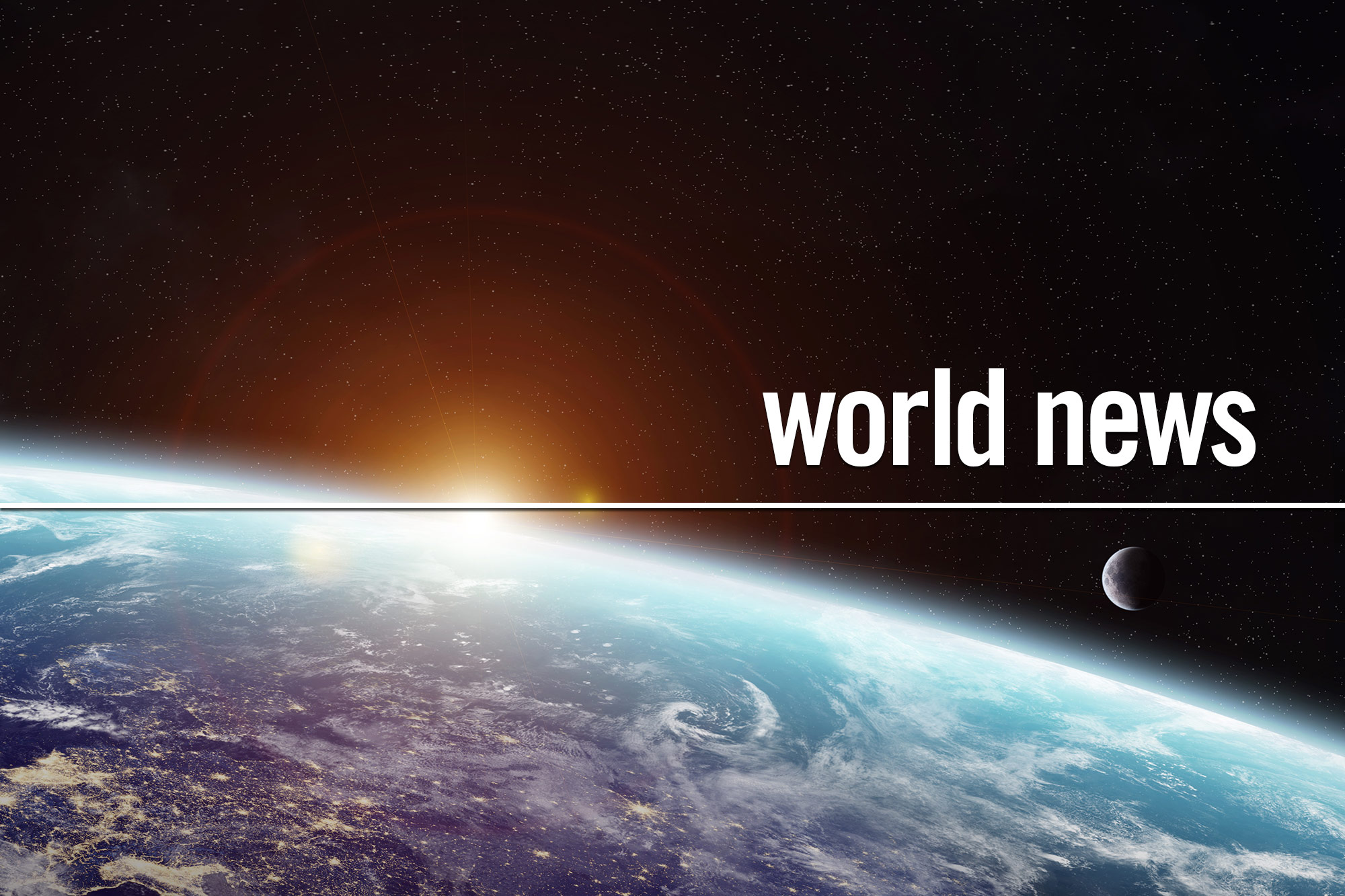A stunning rectangular image showcases a breathtaking view of the Earth captured from a satellite orbiting in space. The top portion is dominated by a vast expanse of a star-studded black sky. As the scene progresses downward, the magnificent curvature of the Earth takes form, stretching from the middle left to the bottom right of the frame. The Earth is partially illuminated by the Sun, which is just beginning to peek over the planet’s horizon on the left-hand side, casting a radiant glow.

In the bottom right corner, the Moon subtly makes its presence known, adding to the celestial beauty of the scene. Cutting through the image is a white line with lowercase text reading "world news," situated prominently in the center. Below this line, the Earth's surface reveals intricate details: swirling cloud formations, vast oceans, and varying landmasses. On the bottom left-hand side, the twinkling lights of a city emerge from the darkened landscape, indicating human habitation in this otherwise serene, out-of-this-world perspective.